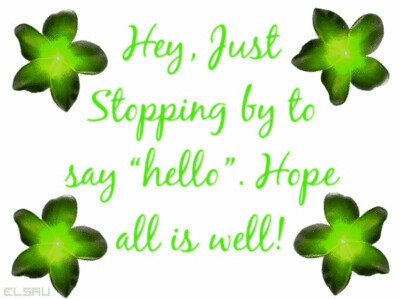The image features a stark white background adorned with four green flowers, one positioned in each corner. Each flower has five petals displaying a gradient from a dark green at the edges, transitioning to a vibrant, neon green at the center. The petals are uniquely varied in shape. At the heart of the image, light green, cursive text reads: "Hey, just stopping by to say 'hello.' Hope all is well!" Each flower appears meticulously detailed with its gradient coloration creating a vivid contrast to the plain background. In the bottom left corner, a light gray watermark reads "E-L-S-A-U," adding a subtle signature to the design. The overall arrangement and color scheme give the image a simple yet charming appearance, resembling a quaint postcard or flyer.